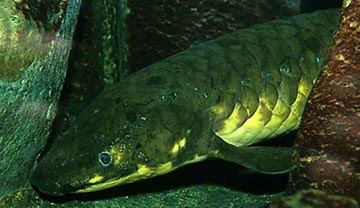This underwater photograph captures a detailed and realistic depiction of a fish, set in what appears to be an outdoor aquatic environment, possibly a pond or an enclosure. The fish, angled at 45 degrees, showcases its distinctive dark green, almost murky upper body and a contrasting light-colored, almost glowing, whitish-green underbelly. Its large, circular scales are clearly visible, emphasizing the contrast between the two sections of its body. The fish's visible eye stands out as a dark blue with a black iris, adding to the sense of realism in the image. To the right of the fish, a dark purple rock is visible, while the left side features a gray rock, contributing to the natural atmosphere. The surrounding water is notably murky, indicating a potentially shaded or less illuminated environment. The fish's small fin, oriented toward the viewer, suggests it is a slow-moving, cold-water species, rather than a fast, agile tropical fish.